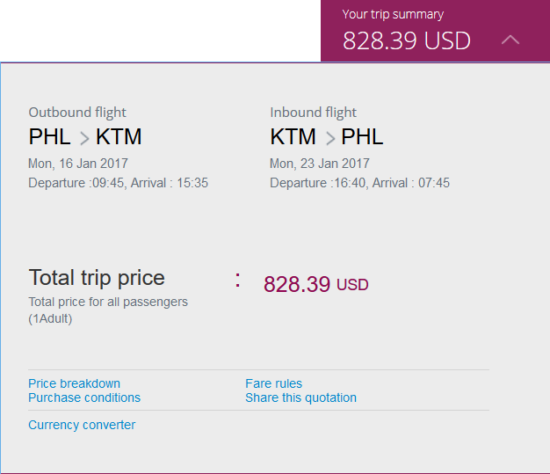Detailed caption:

"Trip Summary for Tom Pratt shows a total cost of $828.39 USD. The image contains a purple square followed by a line, adjacent to a gray square featuring detailed text. The text outlines an outbound flight from Philadelphia (PHL) to Kathmandu (KTM) scheduled for Monday, January 16th, 2017, with a departure time of 9:45 AM and an arrival time of 3:35 PM. Additionally, there is information about the inbound flight from Kathmandu (KTM) back to Philadelphia (PHL) on Monday, January 23rd, 2017, departing at 4:40 PM and arriving at 7:45 AM the next day. The total trip cost for one adult is $828.39 USD, which includes a detailed price breakdown and purchase conditions. There's also an option to convert the quotation into different currencies and share the details. The text also features repeated references to the route and cost, emphasizing important information such as flight details and pricing."